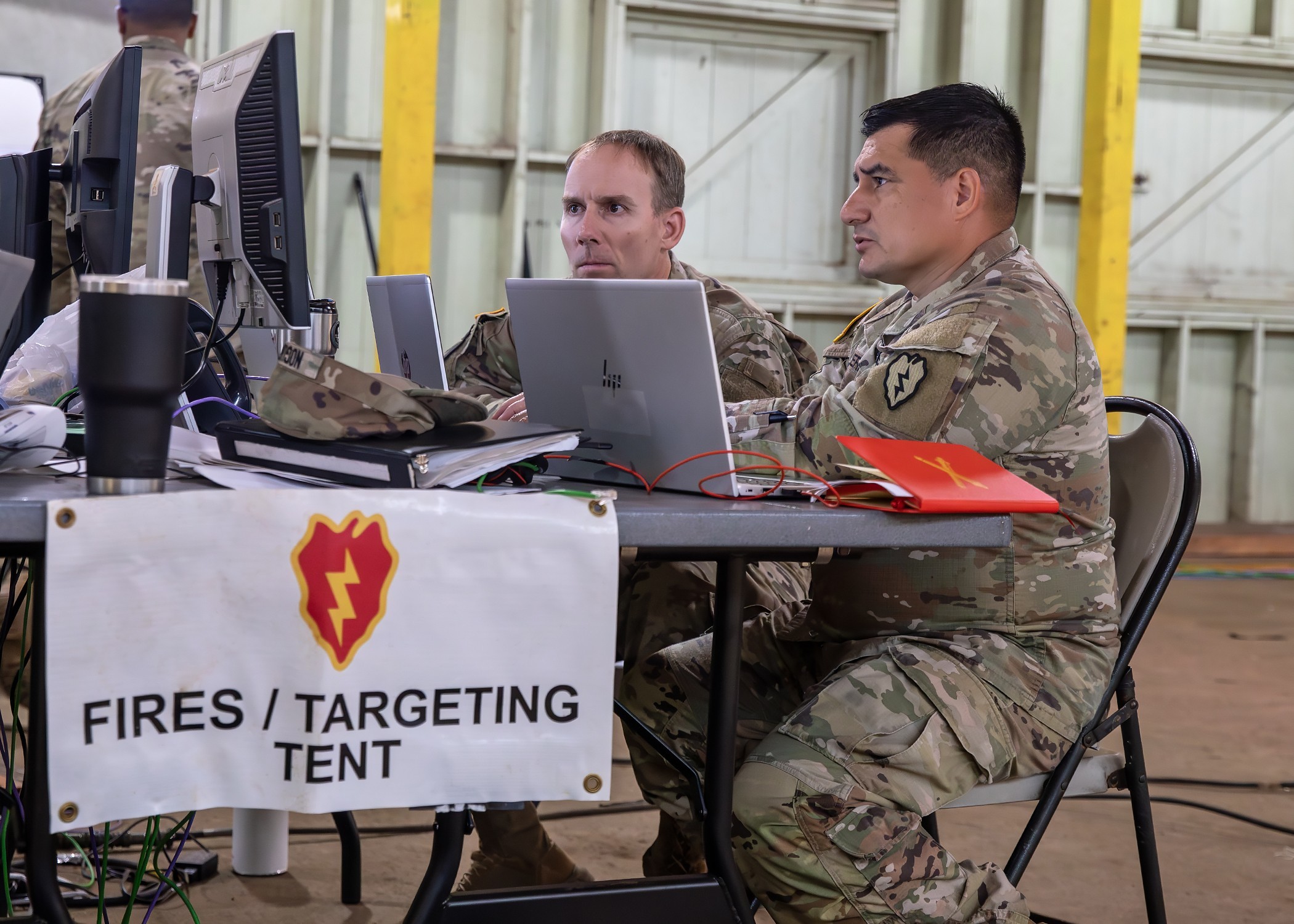The photograph shows two men in army fatigues sitting at a folding table with dark legs and a gray tabletop, both engrossed in their respective HP laptops. The man on the left has light brown, receding hair and light skin, while the man on the right, with darker, almost black hair, has tanned skin, suggesting he may be of Italian or Hispanic descent. The table is adorned with a white banner that bears the black text "FIRES-TARGETING TENT" alongside a red flame logo. In addition to the laptops, there are a couple of desktop monitors positioned behind them on the left side of the table. Beside the man with dark hair sits a red folder, and behind his laptop, a camouflage hat rests on a binder. The setting includes a light brown ground, possibly indicating a military environment, with sturdy military doors or entranceways visible in the background.